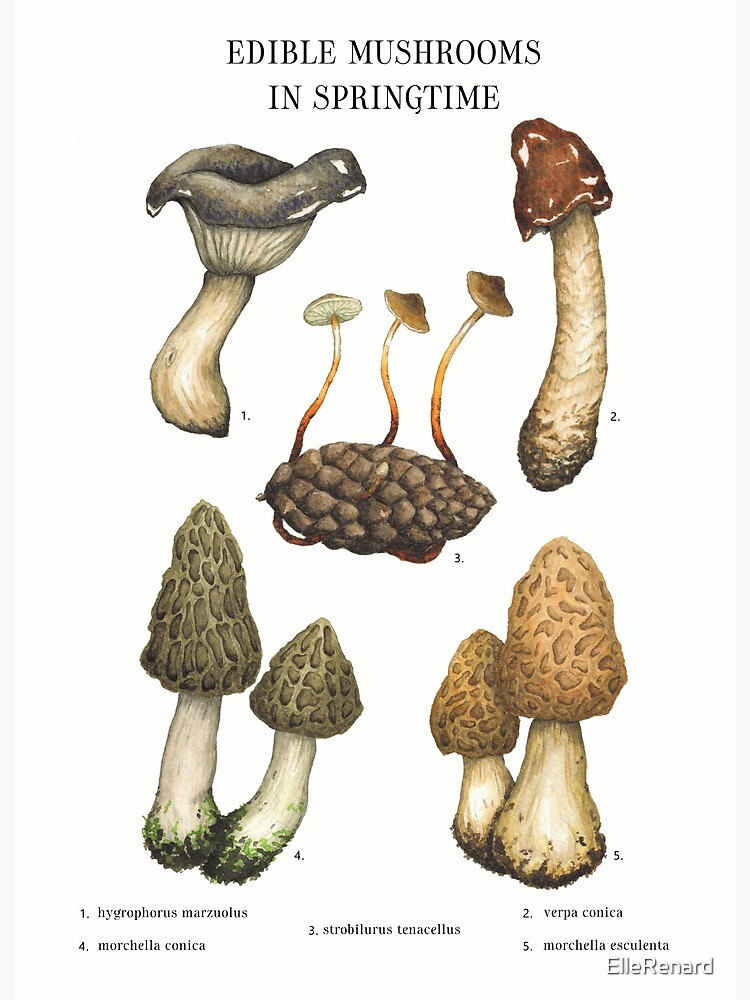The infographic titled "Edible Mushrooms in Springtime" presents a detailed and colorful illustration of five different types of edible mushrooms against a light gray background. The title is displayed in black serif font at the top. Each mushroom illustration is numbered from 1 to 5, corresponding to detailed descriptions and their scientific names listed at the bottom of the image. 

1. The first mushroom, "Hygrophorus marzolos," features a curved stem and a bowl-shaped cap with an outwardly curved lip.
2. The second mushroom, "Verpa conica," has a tall stem with a cone-shaped red cap.
3. The third mushroom, "Strombolurus tenacilis," resembles a pine cone with long, thin stems and cone-shaped caps, suggesting they might be growing out of the pine cone.
4. The fourth mushroom, "Morchella conica," has a medium-length stem and a gray, textured, cobblestone-like cone-shaped cap.
5. The fifth mushroom, "Morchella esculenta," is similar to the fourth but features a tan color and slightly fatter stems.

At the bottom right corner, the artist's name, L. Renard, is inscribed, adding a signature touch to the detailed and educational visual guide on springtime edible mushrooms.